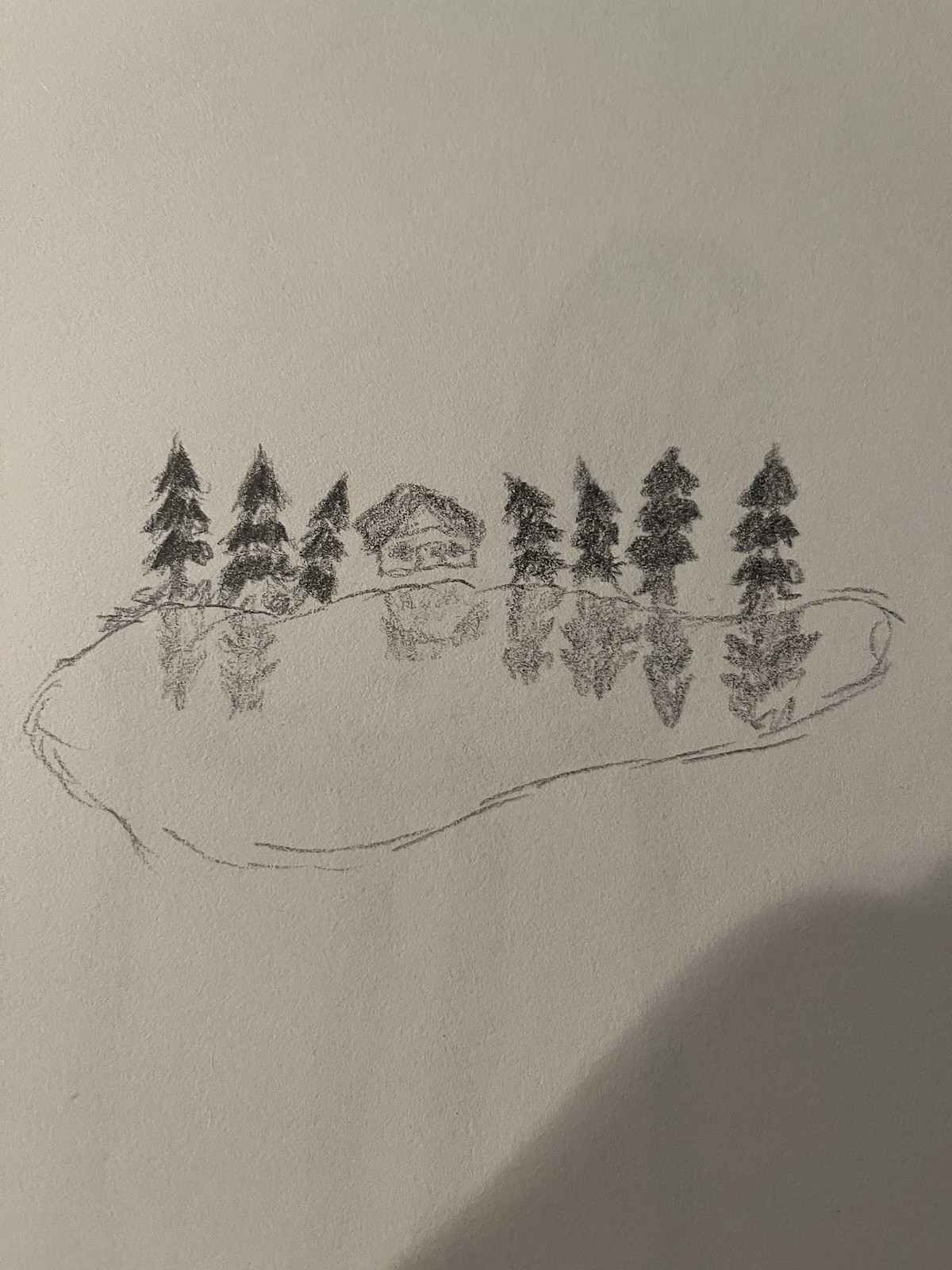This detailed pencil drawing features an oblong lake surrounded by evergreen trees. The artist has intricately sketched each element, though some lines remain deliberately unconnected, lending an artistic texture to the piece. In the middle of the scene, a quaint house stands, perfectly mirrored in the lake’s surface alongside the trees. The reflections are lightly shaded, clearly marking them as reflections. A shadow encompasses the lower right-hand corner of the image, adding depth and dimension. Additionally, a faint impression of a four-legged creature, possibly a dog or a horse, has bled through from the opposite side of the paper, subtly visible as a shadowy silhouette against the serene lakeside scene.